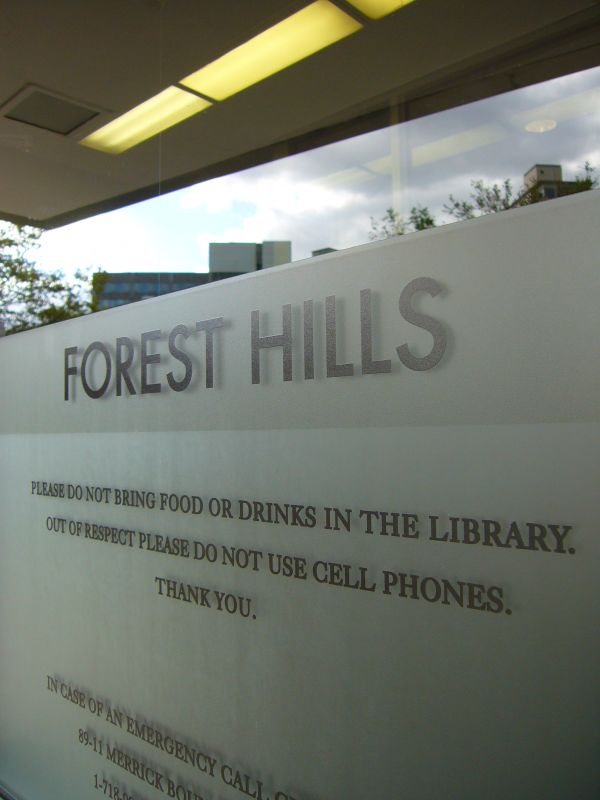This photograph captures the exterior of a modern, glass-fronted building named "Forest Hills." The glass facade is remarkably clear and well-maintained, reflecting surrounding buildings and ceiling lights. Prominently displayed on a gray, marble-like sign beneath the windows, the building’s name, "Forest Hills," is written in all capital letters. Below this title, a set of guidelines is provided for patrons, requesting, "Please do not bring food or drinks in the library. Out of respect, please do not use cell phones. Thank you." Further down the sign, partially visible text begins with, "In case of emergency, call," followed by cut-off information likely meant to include an emergency contact number and additional details. This signage, alongside the architectural features, suggests that the building is a library, possibly associated with a university or other educational institution.